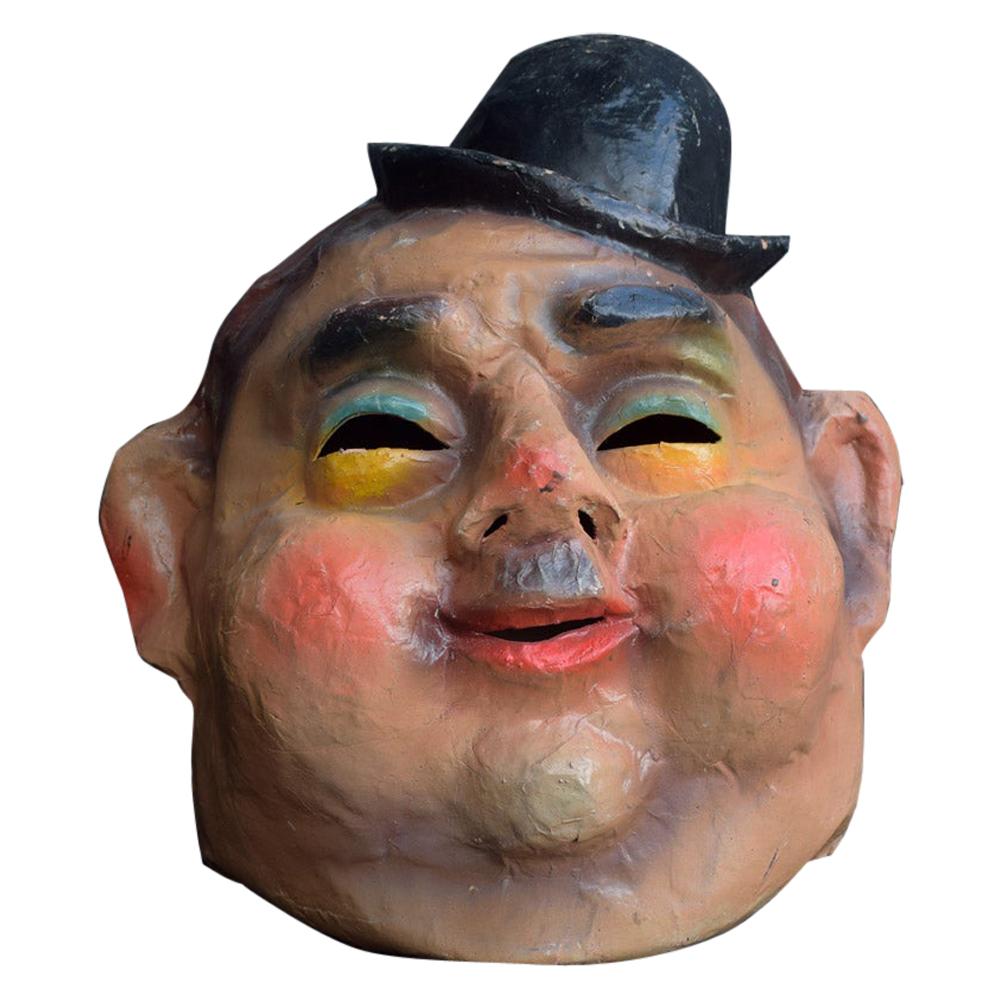The image depicts a ceramic or paper mache mask of an obese, jovial man with a light white complexion. This character, adorned with rainbow-style makeup, prominently features rosy cheeks, a double chin, and a small black hat perched on his head. His eyes are merely openings, revealing the hollow, dark interior of the piece, and the makeup consists of a golden yellow shade below the eyes and a lighter blue above, complemented by very thick, bushy eyebrows. He has a buzz cut or shaved head, big ears, bushy eyebrows, and is sporting an open smile with lipstick on his mouth. His nose is flared and rosy, and there's a hint of stubble near his chin. The mask shows signs of moderate wear, with visible cracks and wear in the pastel painting. Overall, the expression of the man is joyful and friendly.